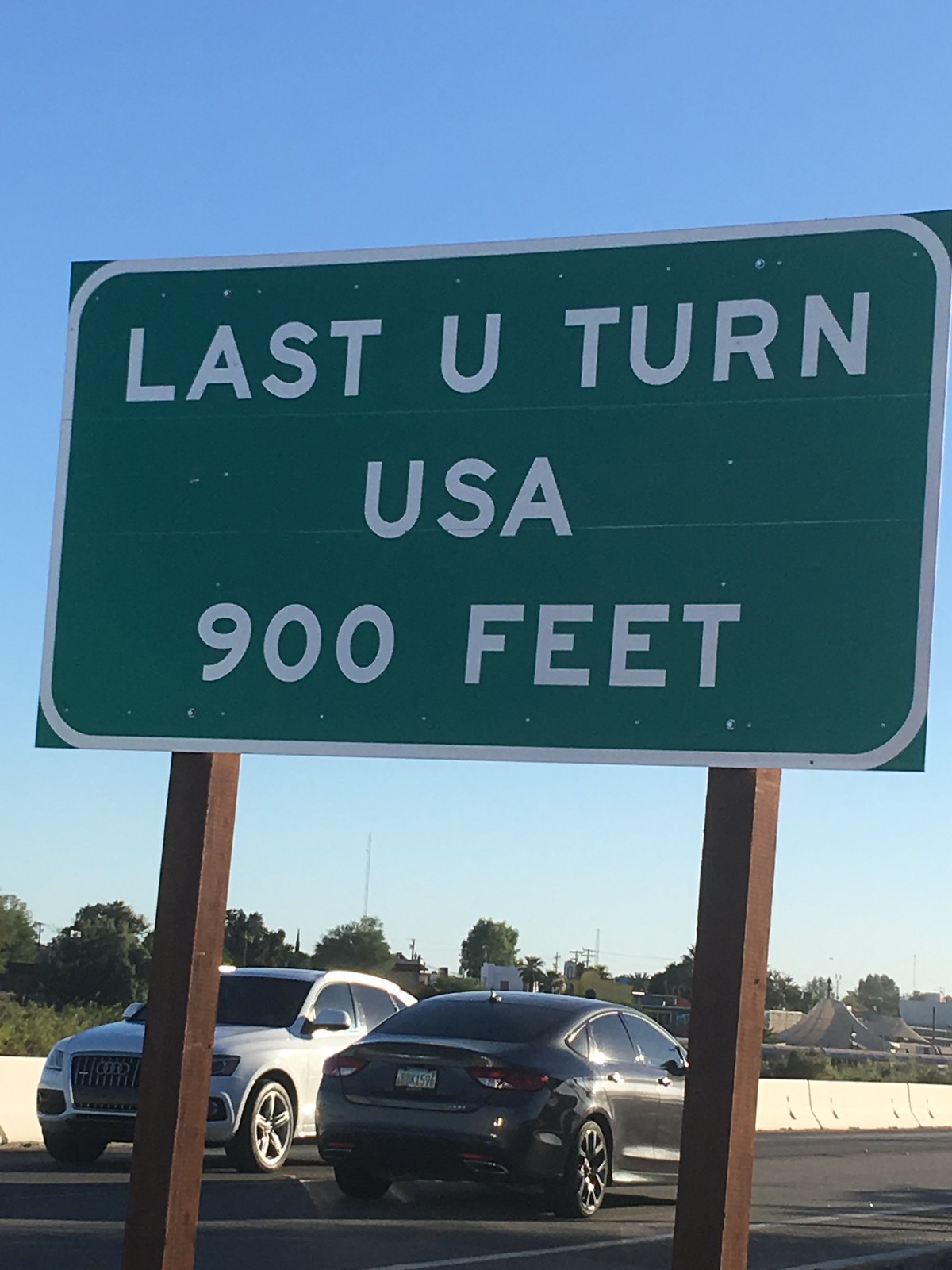The photograph captures a vibrant scene along the side of a highway, distinguished by a prominent highway sign as its focal point. The sign, mounted on two brown, square-shaped wooden posts, features a green panel with a white border, adorned with white text that reads, "Last U-Turn, USA, 900 feet." The black asphalt road stretches ahead, with two cars in motion – a gray car heading in one direction and a silver car traveling in the opposite direction. Sunlight glimmers off both vehicles, enhancing their metallic hues. To the left side of the road, a white barricade is visible. The backdrop showcases a clear blue sky, dotted with a tree line that stretches into the horizon, adding a touch of natural beauty to the scene.